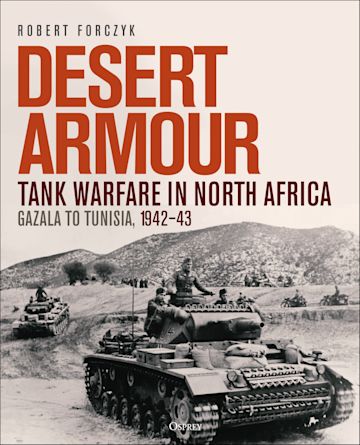The image appears to be the front cover of a book or possibly a movie poster, predominantly in black and white. At the very top, in bold black letters, it says "Robert Forsyth." Below this, in prominent red letters, it reads "Desert Armor." Underneath, in a dark maroon color, the text says "Tank Warfare in North Africa." Further down, in gray letters, it states "Gazala to Tunisia," followed by "1942 to 1943" in maroon. The central image features a black and white depiction of a rugged hillside with brush, dirt, or sand. In the foreground, there is a tank with three men visible on top. One man is wearing what appears to be a gray hat, possibly indicating a captain. Behind this tank, another tank is partially visible, along with at least two motorcycles further in the background, each ridden by a soldier. The composition of tanks, motorcycles, and soldiers emphasizes the wartime setting in North Africa during the specified years, framing the cover's evocative and historical elements.